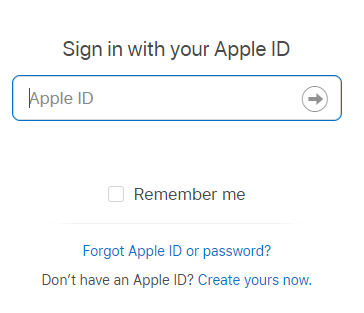A screen capture displays a basic pop-up window prompting the user to sign in with their Apple ID. At the top of the window, a text field is highlighted with a blinking cursor, ready for the user to enter their Apple ID. Directly beneath this field, a label indicates "Apple ID." An arrow icon, positioned to the right of the text field, signifies where users can click to log in after entering their credentials. Below the sign-in field, a checkbox option labeled "Remember me" is available, allowing users to save their login details for future sessions. For those who do not yet have an Apple ID, a hyperlink offers the option to "Create yours now." Additionally, another hyperlink, "Forgot Apple ID or password?", directs users to a page where they can recover their Apple ID by entering their email or reset their password if forgotten. This familiar interface is likely encountered by countless users globally every day.